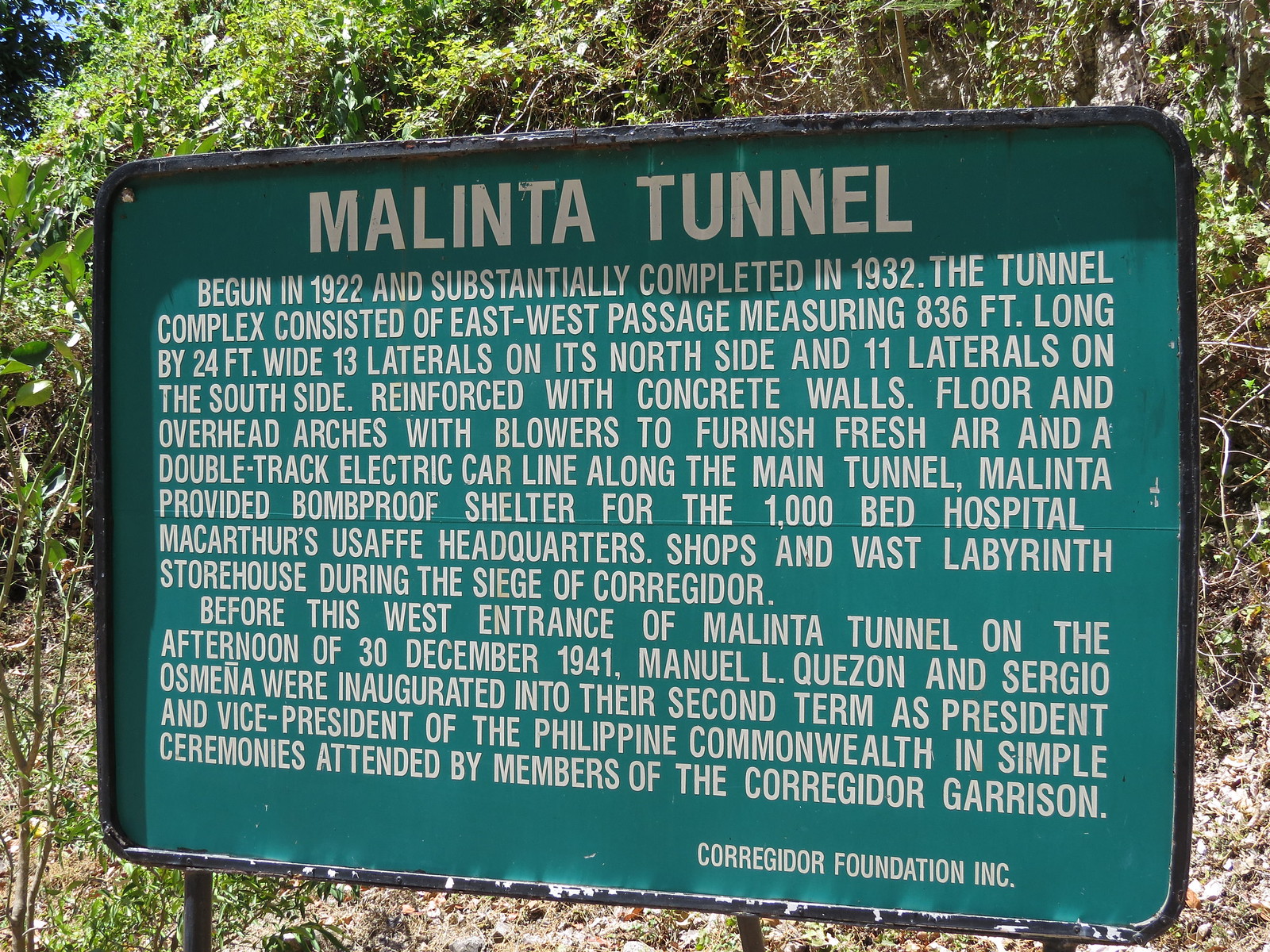This outdoor daytime photograph captures a large green sign with a black border, prominently displaying historical details about the Malinta Tunnel. The sign, which occupies the majority of the frame, presents a perspective where the right side is closer to the viewer, while the left side recedes, revealing a hillside adorned with thin trees and green foliage in the background.

At the top center of the sign, in bold white text, it reads "Malinta Tunnel.” Below that, it states, "Begun in 1922 and substantially completed in 1932." The text continues, detailing that the tunnel complex consists of an east-west passage measuring 836 feet long by 24 feet wide, with 13 laterals on the north side and 11 laterals on the south side. The structure is reinforced with concrete walls, floors, and overhead arches, equipped with blowers to provide fresh air, and features a double-track electric car line running throughout the main tunnel.

The Malinta Tunnel served as a bomb-proof shelter, housing a 1,000-bed hospital, MacArthur's USAFFE headquarters, shops, and a vast labyrinthine storehouse during the siege of Corregidor. Additionally, the sign mentions the historical event on the afternoon of December 30, 1941, when Manuel L. Quezon and Sergio Osmeña were inaugurated into their second term as President and Vice President of the Philippine Commonwealth in a ceremony attended by members of the Corregidor Garrison, held before the west entrance of Malinta Tunnel.

In the lower right corner of the sign, it is noted that this information is provided by the Corregidor Foundation Inc.